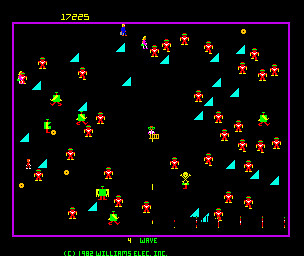This screenshot captures a classic 1982 arcade game developed by Williams Electronic Incorporated. Displayed in low resolution, characteristic of early 1980s technology, the game features a two-dimensional, retro style reminiscent of Pac-Man. The gameplay screen, encased in a purple-bordered frame, reveals a black background dotted with scattered blue triangles. 

At the top left, the player’s score is prominently displayed in yellow, reading 17,225 points, along with "WAVE 4" indicated in green text. Various characters populate the screen – red-outfitted figures with distinct arms, legs, and heads, mixed with other figures sporting green bodies and red legs. These characters seem to be moving in different directions, suggesting an objective to navigate past them to survive.

The green lettering at the bottom reinforces the game's vintage origins, reading "1982 Williams Electronic Incorporated". This old-school video game, likely played on an Atari system, illustrates the early era of digital entertainment with simple graphics and straightforward objectives.